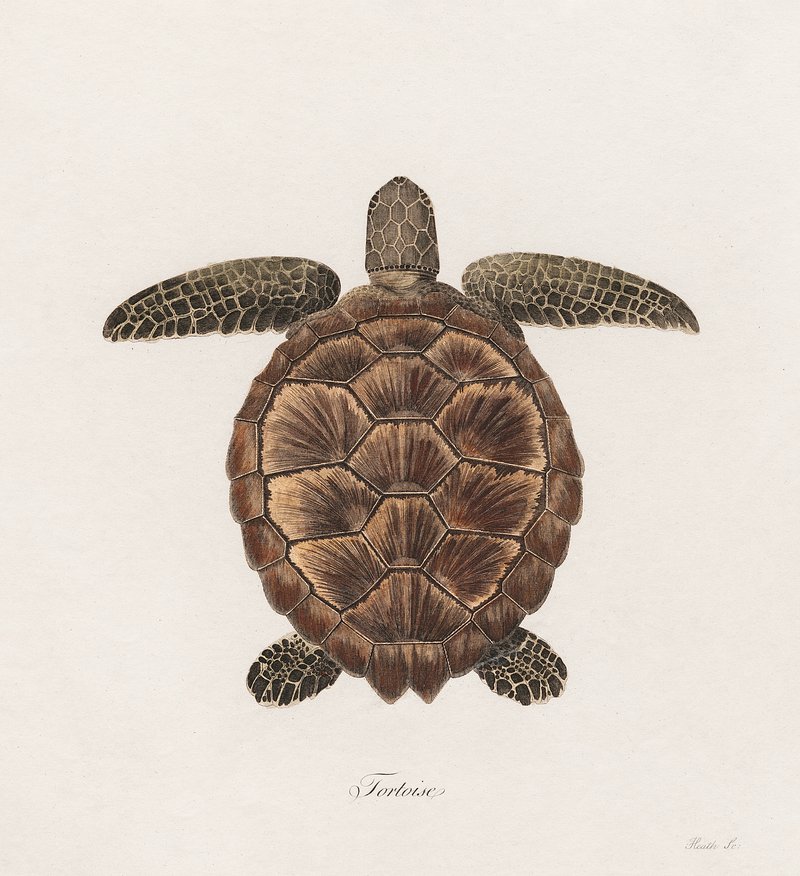The image is a detailed drawing of a tortoise set against a light purple background. The artwork appears to be almost perfectly square, though it leans slightly towards a portrait orientation where the top and bottom edges are shorter than the sides. Centered in the composition is a top-down view of a brown tortoise, showcasing its entire shell, the tops of its front and back feet, and the top of its head. The shell displays a rich brown color with a pattern that resembles a fan or puzzle, interspersed with lighter beige or yellowish tones. The tortoise's head and limbs, which extend outwards, reveal a scaly texture with a mix of blacks, creams, and off-whites, creating a checked appearance. Below the tortoise, in elegant cursive, the word "tortoise" is inscribed. Additionally, there is a faint, small signature in the lower right hand corner of the image.